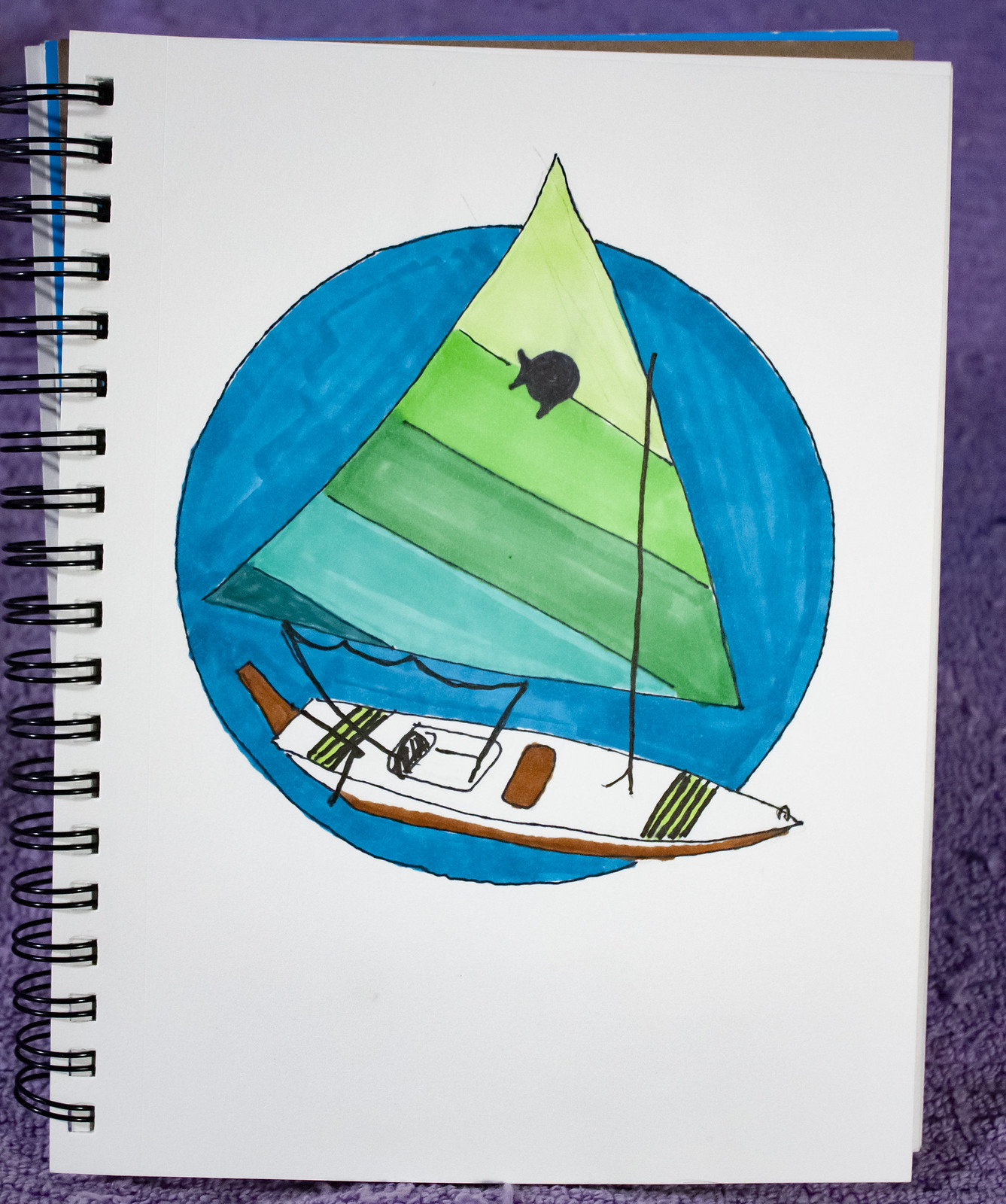A black spiral-bound art notebook rests on a purple-blue towel. The notebook is open and folded back to display a single, detailed ink drawing. The artwork features a boat, resembling a canoe with a sail, encased within a circular frame. The sail, adorned with green and blue stripes, is triangular in shape. The boat itself is depicted with a white and brown hull, accented by small black and yellow stripes. The intricate design highlights the artist's attention to color and form.